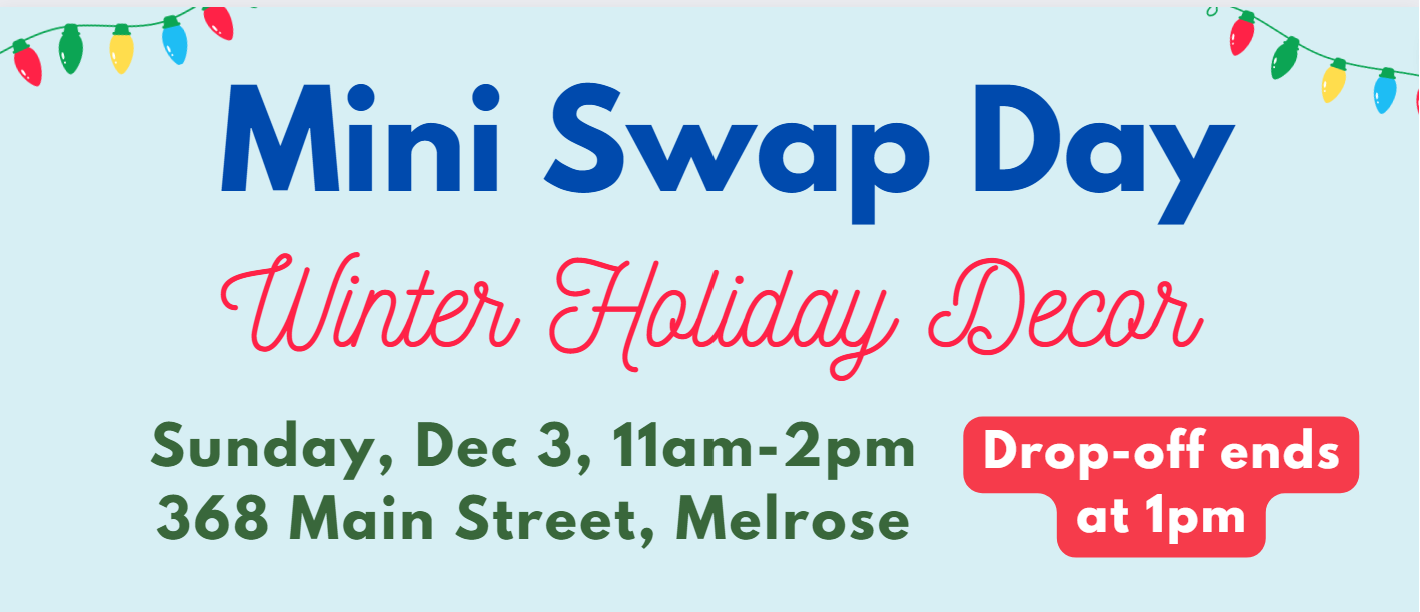This rectangular advertisement image features a light teal background and festive Christmas light illustrations with red, green, yellow, and blue bulbs adorning the top left and right corners. Bold, blue text at the top reads "Mini Swap Day," followed by an ornate red script announcing "Winter Holiday Decor." Below this, green text details the event: "Sunday, December 3rd, 11 a.m. to 2 p.m.," taking place at "368 Main Street, Melrose." In the bottom right corner, a red-bordered text box with bold white letters states, "Drop-off ends at 1 p.m." The blend of colors and festive decorations emphasizes this as a promotion for a community event centered around holiday decor and swapping items.